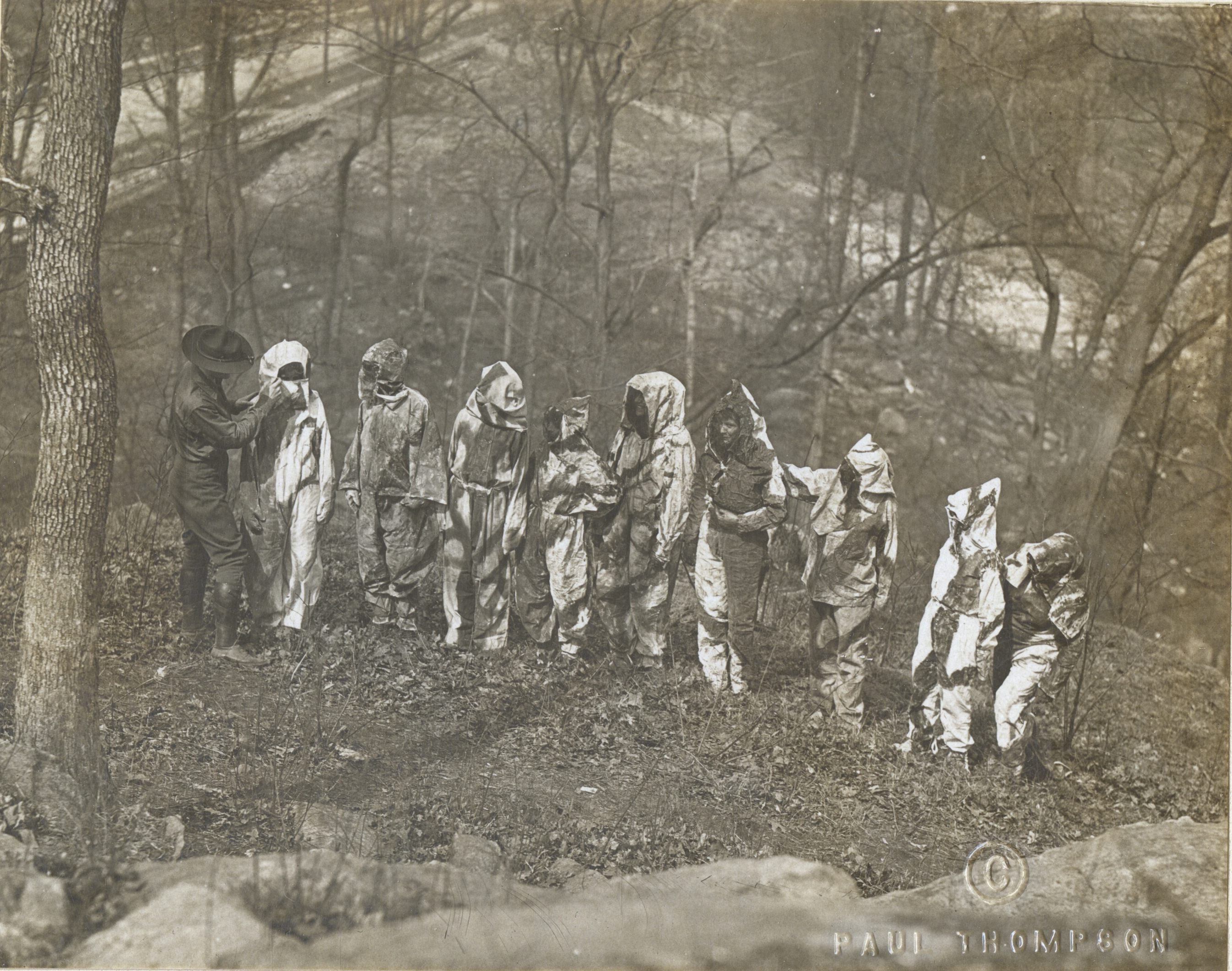This sepia-toned photograph, credited to Paul Thompson in the bottom right corner, depicts a surreal scene in a barren, forested area, likely during the fall or winter months. At the forefront stands a man in what appears to be a military or ranger uniform, complete with high boots, black pants, black shirt, and a hat with a brim. He is adjusting the hood or face covering of the first person in a line of ten individuals. These individuals are clad in oversized, white protective suits that cover them from head to toe, including their faces, making the exact purpose of their clothing ambiguous—ranging from military training to beekeeping or even firefighting gear. The forest is thick with leafless trees, and a road is faintly visible in the top left corner, adding to the eerie, almost otherworldly atmosphere of the scene.